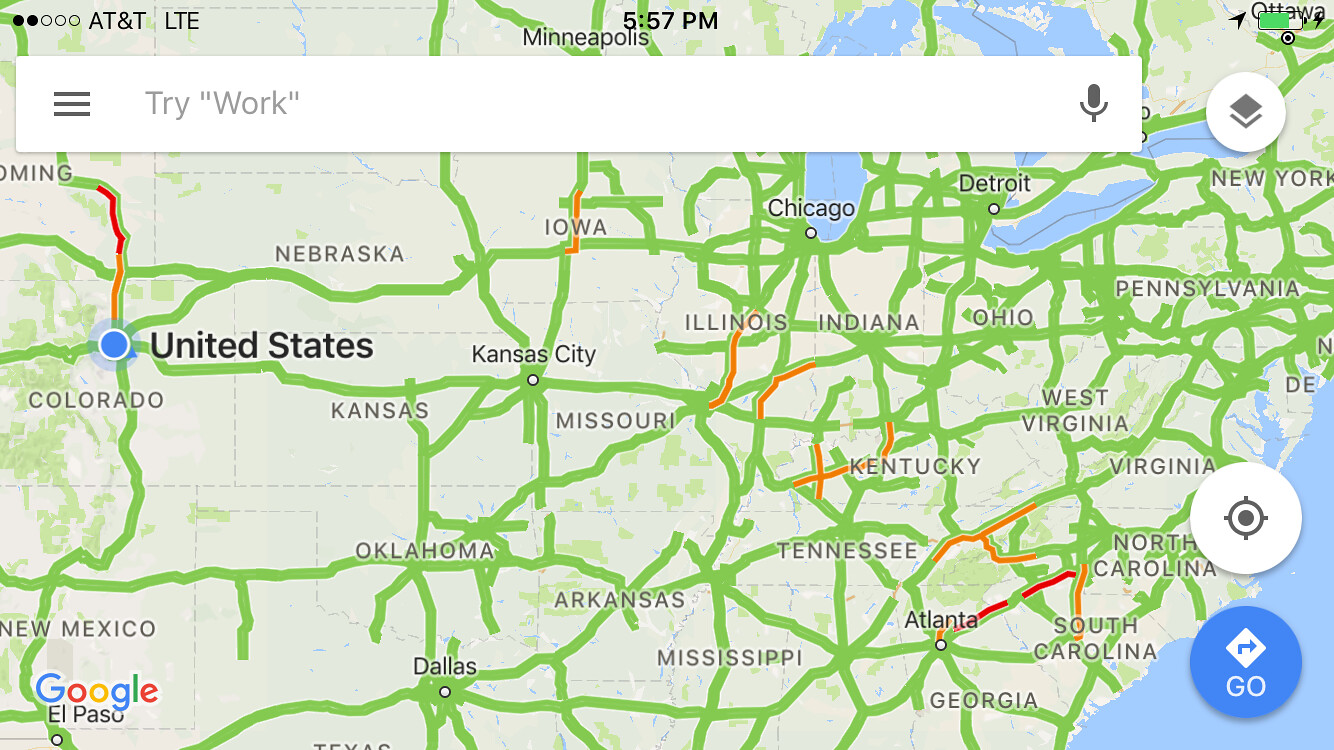This is an image of a map covering a significant portion of the United States with a distinct white background. At the top of the image, there's a white bar where the words "try and work" are displayed with "work" in parentheses and a microphone symbol on the left side. Above this bar, on the left, it states "AT&T LTE" and the time "5:57 PM". The location "Minneapolis" is also mentioned in the center of this top section. 

The map showcases numerous states such as New York, Pennsylvania, West Virginia, Virginia, North and South Carolina, Georgia, Tennessee, Kentucky, Ohio, Indiana, Illinois, Iowa, Missouri, Arkansas, Mississippi, Oklahoma, Kansas, Nebraska, Colorado, New Mexico, and part of Wyoming. However, Michigan isn't labeled. 

Green lines run horizontally and vertically across the map, connecting various points, but there is no legend to explain what these lines represent. Additionally, there are short orange overlays at about nine different locations on the green lines. In the lower left-hand corner, the Google logo is present, adding to the impression that the map is sourced from Google. Moreover, to the left near Colorado, a blue dot with the label "United States" in bold is noticeable.